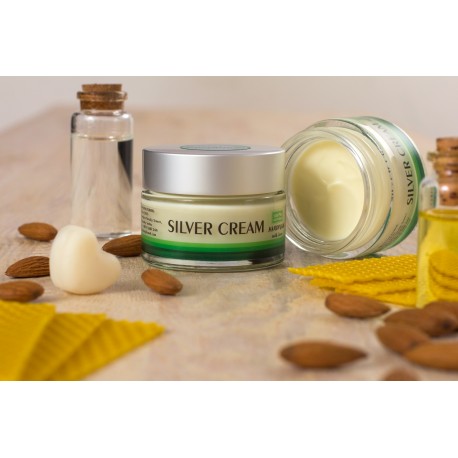The photograph showcases a beige table adorned with multiple items, predominantly featuring jars and bottles. Central to the image is a round glass jar labeled "Silver Cream," distinguished by its silver lid and a decorative band at the base where shades of green transition from light to dark, adorned with horizontal stripes. A similar jar lies on its side nearby, its lid removed to reveal a white-ish yellow cream inside. To the right of these jars is a glass bottle with a yellow fluid, sealed with a cork stopper. Scattered across the table are twelve almonds, adding a natural touch to the scene. Additionally, square yellow items, possibly pieces of honeycomb, and a white heart-shaped object, which appears to be made of wax, are also present, enriching the composition with varied textures and colors.